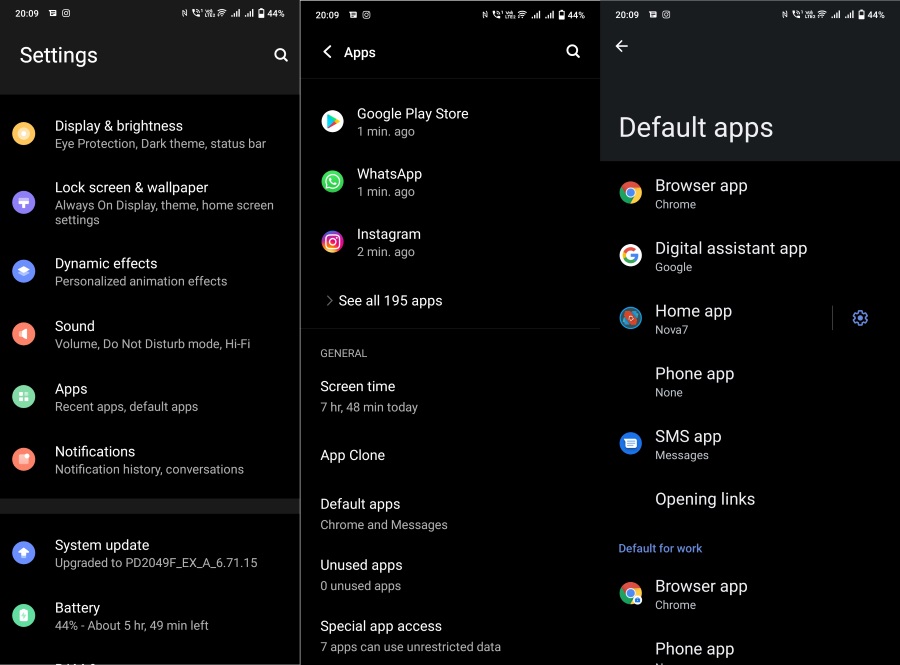The image showcases a computer screen with a predominantly black background, divided into two distinct sections. 

On the left, there is a slim vertical sidebar labeled "Settings". Within this section, there is a small search icon at the top, followed by a list of settings categories, each denoted by a colored circle with an icon. The first category is "Display and Brightness", symbolized by a gold circle. This section includes options such as eye protection, dark theme, and status bar customization. Below this is the "Lock Screen and Wallpaper" category, represented by a paintbrush icon. Other categories follow in the list, each with its own unique colored icon, like "Dynamic Effects", which appears to have a graduation cap icon (although it is somewhat blurry), and "Sound", marked by a red circle with a megaphone icon.

The right side of the screen is significantly larger and continues with the black background theme. This area displays information regarding "Apps and Default Apps". At the top, larger text highlights this section, listing examples of apps such as Google Play Store, WhatsApp, and Instagram. Beneath this, in a slightly larger font, is the "Default Apps" heading. Below it are detailed options for default applications, including categories like Browser app, Digital Assistant app, and Home app, all organized vertically into two rows. This layout offers a comprehensive view of both the customizable settings and default applications available on the system.